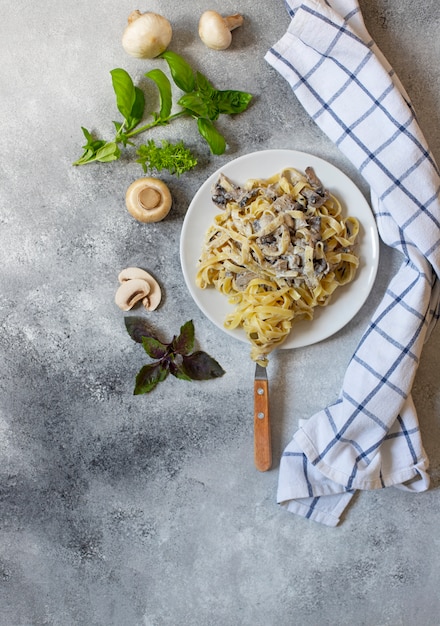The image showcases a beautifully plated dish of Fettuccine Alfredo with mushrooms on a white ceramic plate. The fettuccine is generously coated in a creamy Alfredo sauce and is adorned with slices of mushrooms and an additional unknown topping that may be chicken. A light brown wooden handle fork, with some pasta twirled around it, rests on the plate. Sitting below it, partially hanging off the edge. Surrounding the plate, there are several whole mushrooms scattered alongside sliced mushrooms, adding a rustic touch to the presentation. Fresh greenery, including sprigs of basil and possibly chocolate mint, embellish the scene, enhancing the visual appeal and suggesting freshness. The white plate is complemented by a white and blue striped cloth casually twisted to frame the artful arrangement. The background is a neutral, possibly concrete surface that highlights the vibrant details of the dish, making the presentation both appetizing and visually appealing.